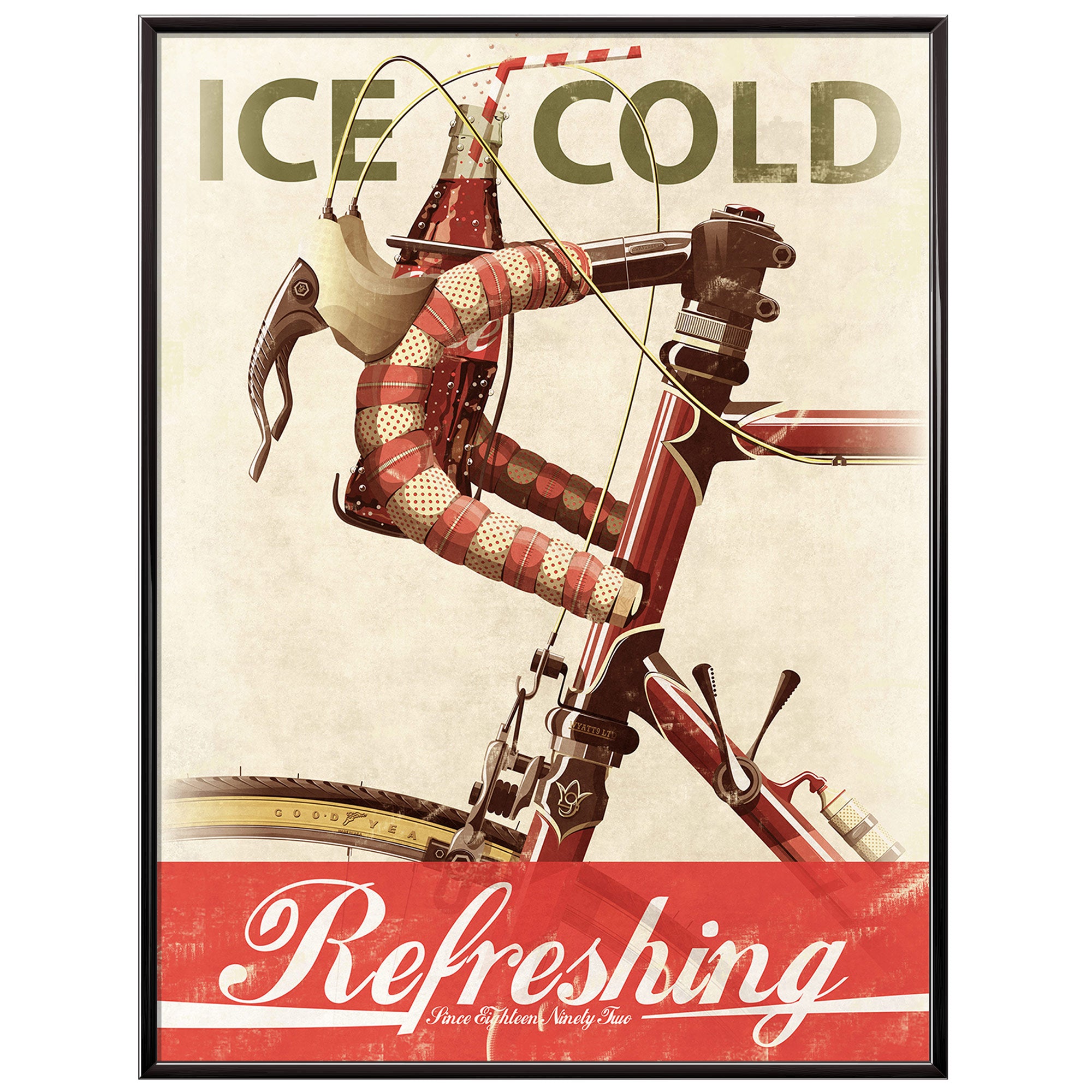This image, rendered in a rectangular 5 to 6 inches high by 4 inches wide format, features a vintage Coca-Cola advertisement encased in a thin black frame. The artwork is set against a light brown, tan, or off-white background. At the top, in an olive green font, the phrase "ice cold" stands out, while at the bottom, framed by a red banner with elegant white cursive, it reads "refreshing" with a tagline indicating "since 1892."

Central to the image is the front view of a red and black racing bicycle, complete with Goodyear tires. The bicycle's handlebars, painted in white and red, support a glass bottle of Coca-Cola adorned with a red and white striped straw, slightly bent at the top. The glass bottle showcases a dark brown liquid, typical of Coke, with visible condensation, imparting a refreshing, retro aesthetic to the overall scene.